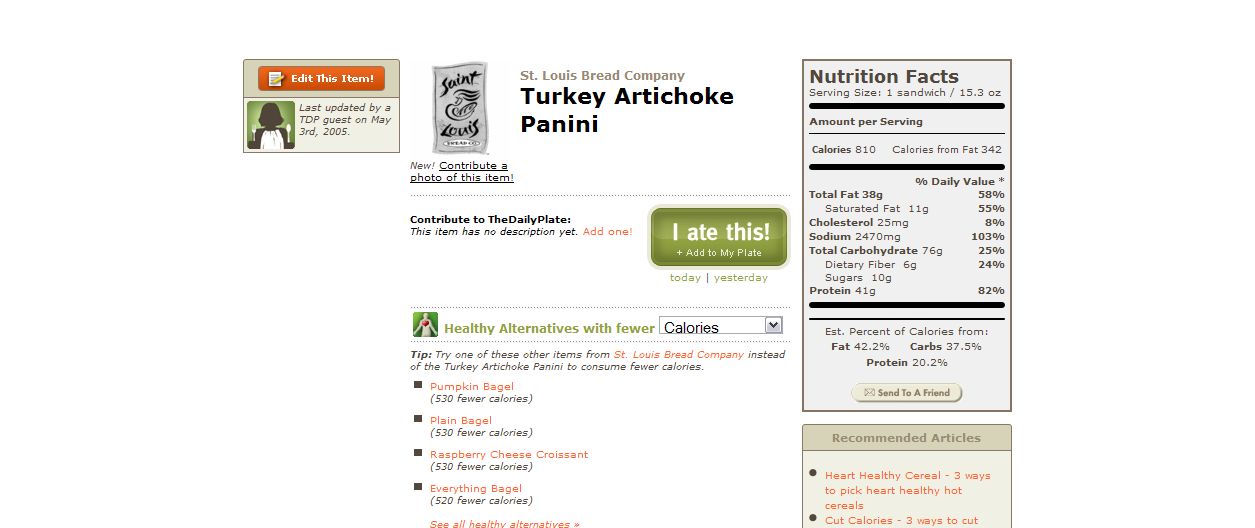The screenshot showcases detailed nutritional information for a Turkey Artichoke Panini, produced by the St. Louis Bread Company. At the top, the company name and logo are clearly visible on the left side. On the right side, the nutrition facts are presented with fine print. The panini contains either 610 or 810 calories, with a higher likelihood of 810 calories due to the significant quantities of nutrients listed: 38 grams of fat (including 11 grams of saturated fat), 76 grams of carbohydrates, 41 grams of protein, and 10 grams of sugar. Central to the image is a section highlighting healthier alternatives with fewer calories. This part lists four items: Pumpernickel Bagel, Plain Bagel, Raspberry Cheese Croissant, and Everything Bagel, all of which have calories ranging from 500 to 600, significantly less than the presumed 810 calories of the panini.